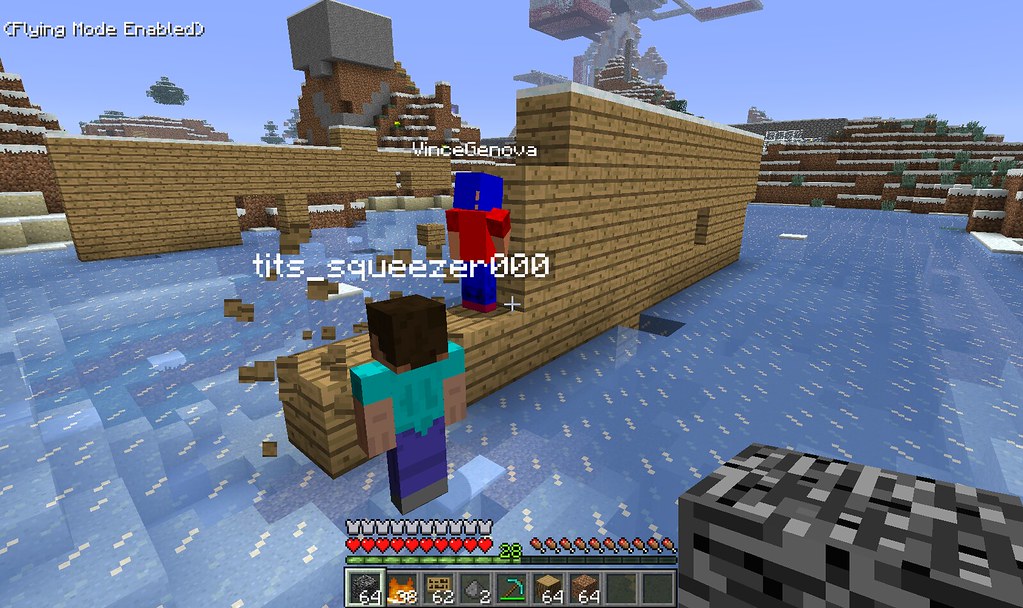The image is a colorful screenshot from Minecraft, capturing a lively in-game moment. The scene is depicted from a player's first-person perspective, showcasing their inventory filled with stone, wood, a diamond pickaxe, coal, fire, signs, and crafting tables. Notably, a humorous username, "SomethingSqueezer000," appears over a character sporting the default Steve skin. He seems to be collaborating with another character named "Vince Genova," likely a nod to Final Fantasy 7, as they work on constructing a building or setting up wooden structures. The background reveals an incomplete brick wall in front of a blue sky, indicating an ongoing building mission. To highlight the gameplay aspects, the text "Flying mode enabled" is displayed at the top, adding to the dynamic nature of the scene.